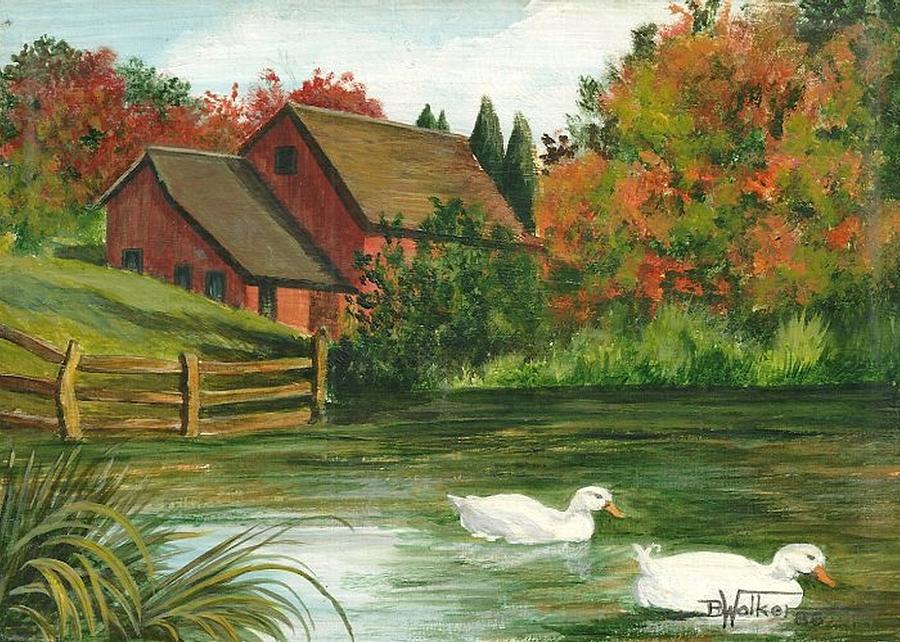This is an oil painting by B. Walker, likely created in 1985, depicting a serene farm scene in the autumn. In the foreground, two white ducks with orange bills swim gracefully in a pond, their movement creating ripples in the water. Surrounding the pond are lush patches of green grass and a brown fence with slats stretching towards the left, where a green bush thrives. The left side of the painting features a rolling hill topped with vibrant fall foliage in shades of red, green, and orange. Atop this hill, slightly obscured by the trees, stands a red barn-like building with a brown roof and several windows, its paint weathered to a dull red. Behind the barn, more trees in varying autumnal hues stretch across the landscape, against a sky of light blue with wispy white clouds. The painter's signature, "B. Walker '85," is inscribed in black at the bottom right corner.